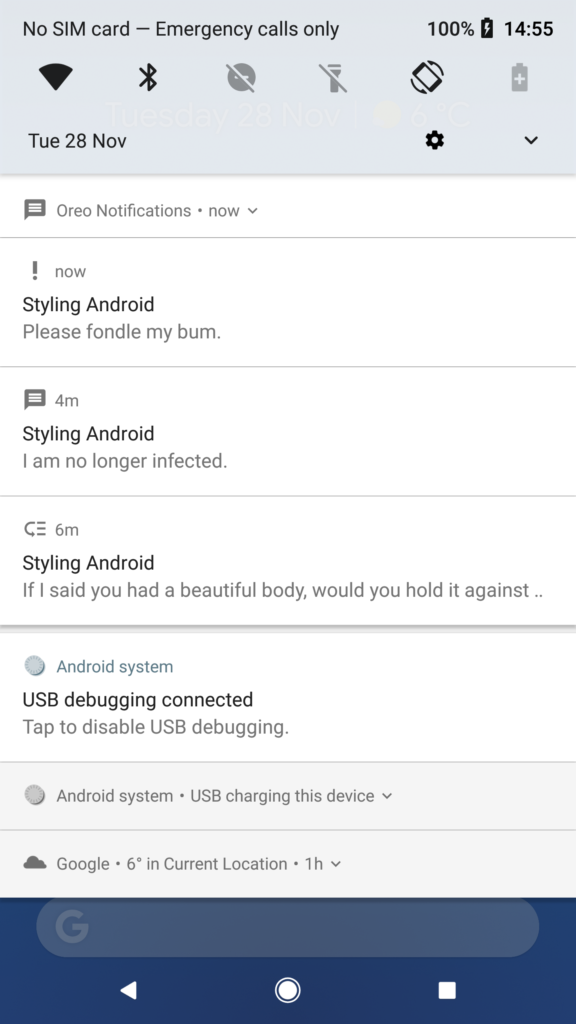The top section of the phone's notification screen features a gray status bar that spans across its width. This bar includes a series of icons from left to right: the signal strength indicator for the phone, Wi-Fi, Bluetooth, a circle with a minus sign to denote 'Do Not Disturb' mode, a crossed-out torch icon, screen rotation lock, and a battery status icon. Directly below this status bar, on the left side, the date is displayed as "Tue, 28 Nov." On the right side, there is a Settings button along with a dropdown menu button. Below this row, the background reveals a list of four notifications.